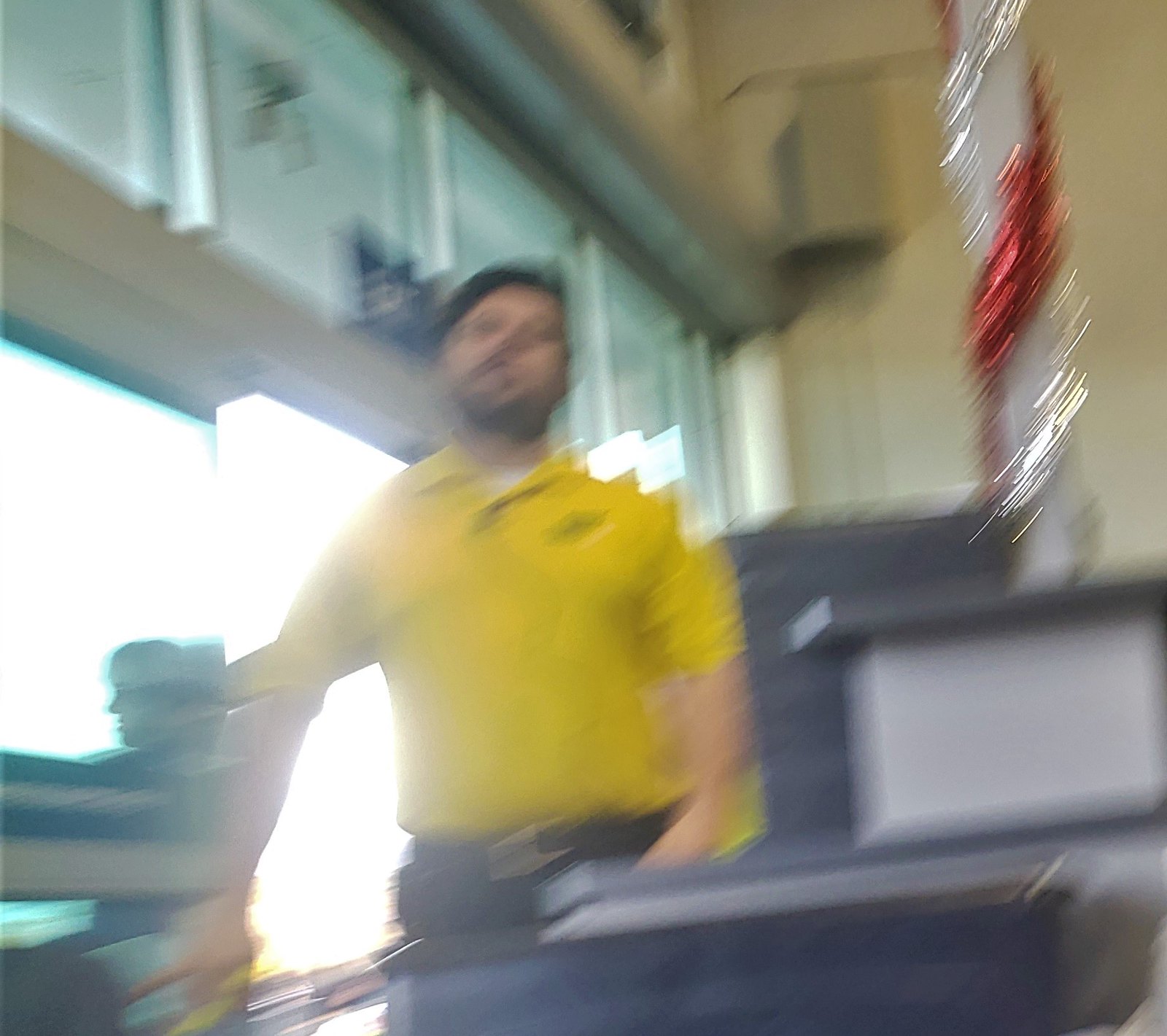In this slightly blurry color photograph, a gentleman with dark hair and a beard is depicted standing inside a building. He is wearing a yellow polo shirt adorned with an indistinct logo on the pocket area. Sunlight from outside illuminates the scene, streaming through glass windows positioned above and to the right of the man. Additionally, another figure is present to the right of the gentleman, though this person is also blurred and their details are indistinct.

Overhead, bright red and silvery decorations, reminiscent of Christmas ornaments and vintage silver tinsel garlands, hang from a white post, adding a festive atmosphere to the scene. In the background, a beige-colored tile wall is partially visible, further defining the indoor setting of this photograph.